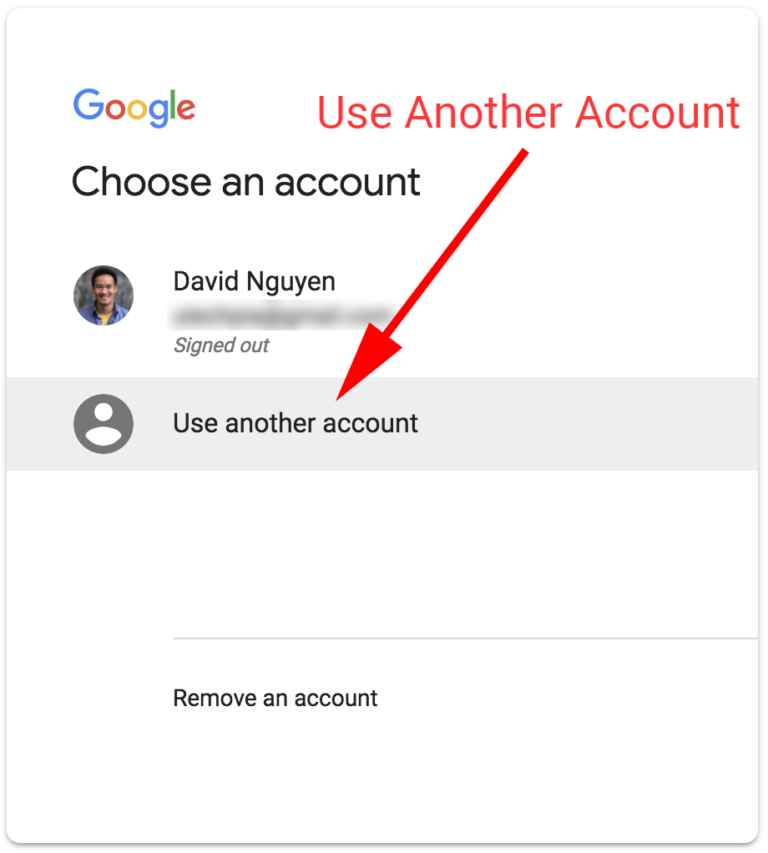**Image Description:**

Category: Websites

The image showcases a simple login interface presumably from Google's account sign-in page. The main section is a white rectangular box outlined with a grey border. 

**Top Section:**
- On the top left, the Google logo is displayed with each letter in its iconic colors: "G" (blue), "o" (red), "o" (yellow), "g" (blue), "l" (green), and "e" (red).
- To the right of the logo, large red text states "Use another account." An arrow points downward towards a grey bar below that text. 

**Middle Section:**
- Within the grey bar, a placeholder icon of a generic person indicates the option to use another account.
- Above this grey bar is a profile picture of an Asian man set against a grey background. The man, named "David Nguyen," is wearing a blue shirt and has dark hair. The details of his features are not clearly visible. 
- Below his name, something is blurred out, followed by text indicating that this account is currently signed out.

**Bottom Section:**
- The lower part of the interface includes a white area with the option to "Remove an account" written in black text.

Overall, the letters on the page are predominantly black except for the colored Google logo and the red, prominent "Use another account" text. The layout is clean and minimalistic, focusing primarily on account management options.